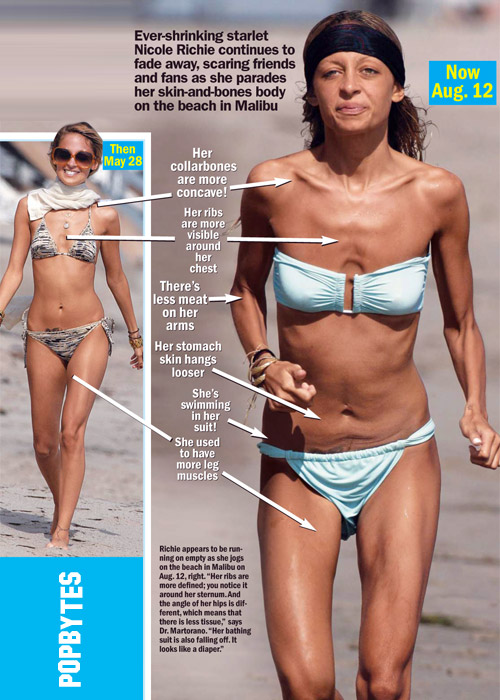The image is a page from a tabloid featuring two photographs of Nicole Richie, juxtaposed to highlight her physical transformation over time. On the left, a smaller picture dated May 28 shows Nicole on the beach in a black and white tiger stripe bikini. On the right, occupying a larger portion of the page and dated August 12, Nicole is depicted in a light blue bikini with a black headband, again on the beach. The captions emphasize her dramatic weight loss, describing her as an "ever-shrinking starlet" with concave collarbones, visible ribs, and looser stomach skin, noting that she appears to be "swimming in her suit." The overall theme of the text is concern from friends and fans due to her increasingly thin appearance. The color palette of the page includes peach, brown, black, white, light blue, greenish teal blue, and yellow, adding to the visual impact. The bottom of the page contains additional unreadable tiny text, reinforcing the article’s dramatic tone.